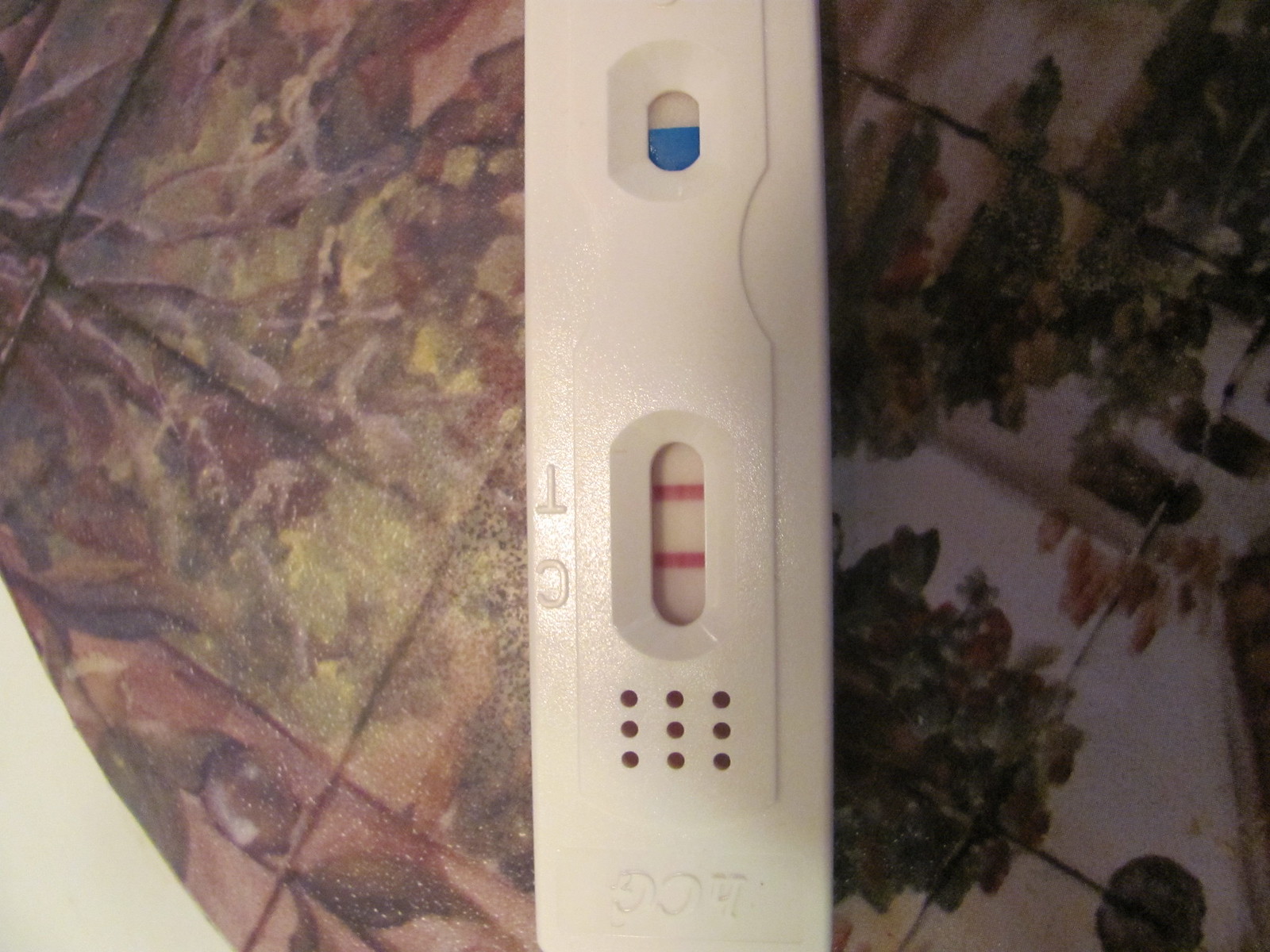This is a close-up photograph of what appears to be a COVID-19 test device. The device is predominantly white and features two distinct test windows. The first, smaller window displays a dual-color indicator, half blue and half white. The second, slightly larger window, situated next to the first, is labeled with 'C' on the top and 'T' on the bottom. This window distinctly shows two red lines, indicating a positive result. Below these windows, there is a series of nine small holes lined up in a grid formation. The test device is placed on a surface that seems to be composed of intricately hand-painted tiles. These tiles are decorated with purple flowers and green foliage against a cream-colored background. The tiles have a rough texture, adding to their artistic, possibly vintage appearance.